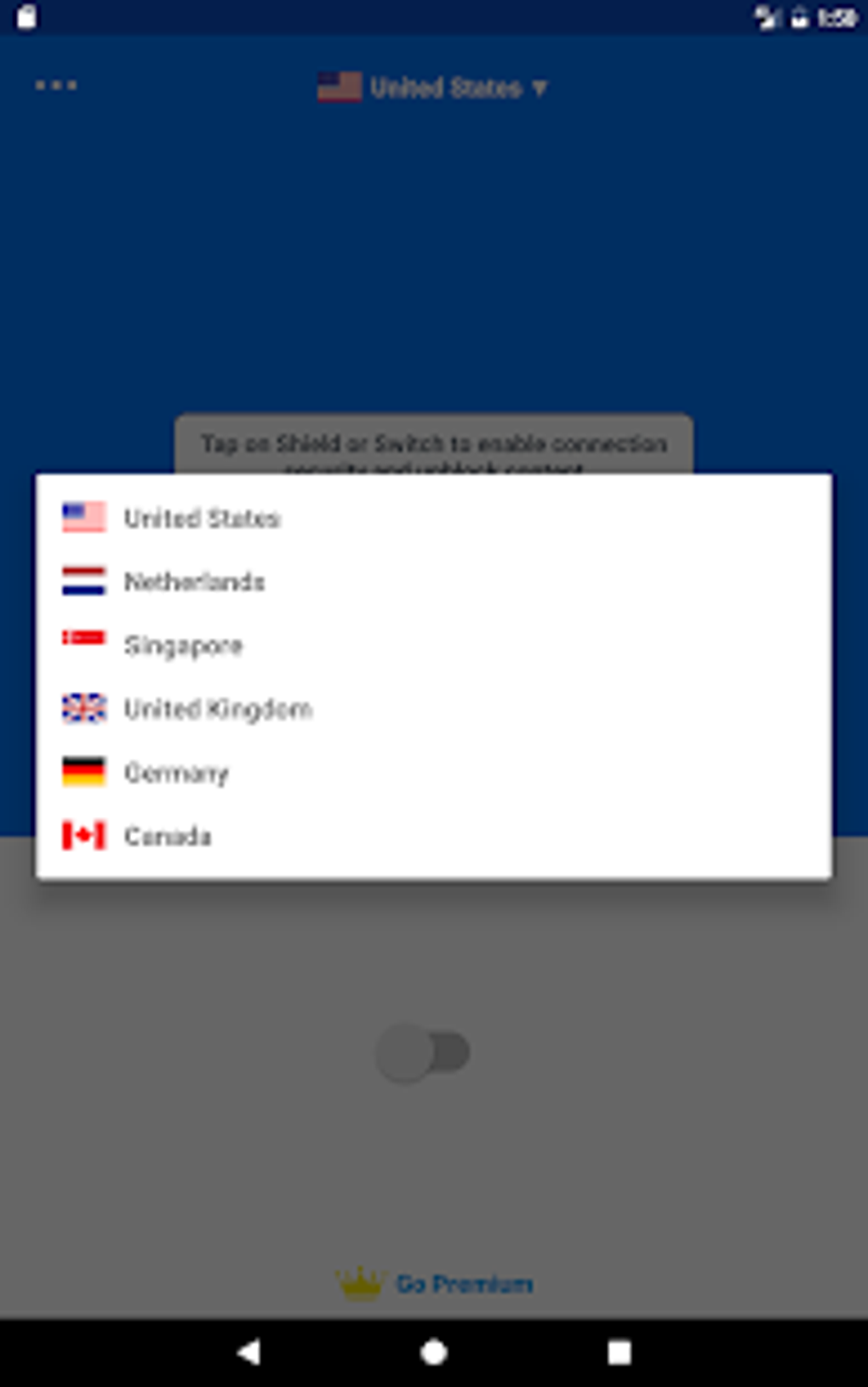This is a screenshot likely taken from a tablet, albeit slightly blurry and out of focus. Near the top of the screen, a dark blue banner spans across with a white icon on the left side. The top right corner of the banner contains three icons, one of which resembles a battery icon, and possibly a time indicator, though it is unreadable due to the blurriness. Beneath this banner, the background shifts to a lighter blue, featuring the word "United States" centered at the top in white letters, accompanied by a red, white, and blue flag to its right. To the left of "United States" are three small dots, and an arrow points downward beside the country's name, suggesting a dropdown menu. 

Below this section, there is a white rectangular box prompting the user with the message: "Tap on shield or switch to enable connections." Subsequently, a window overlays the lighter blue background, displaying a list of countries: United States, Netherlands, Singapore, United Kingdom, Germany, and Canada. Each country name is preceded by its national flag. Within this window, an unlocked white button appears, hinting at functionality related to the listed countries. At the bottom of the window, a yellow crown icon sits beside blue text urging users to "Go Premium." Further down, three buttons are visible, potentially for actions like "Stop" or "Record."

The overall background of the screenshot remains darker and less distinct behind this prominent rectangular window.